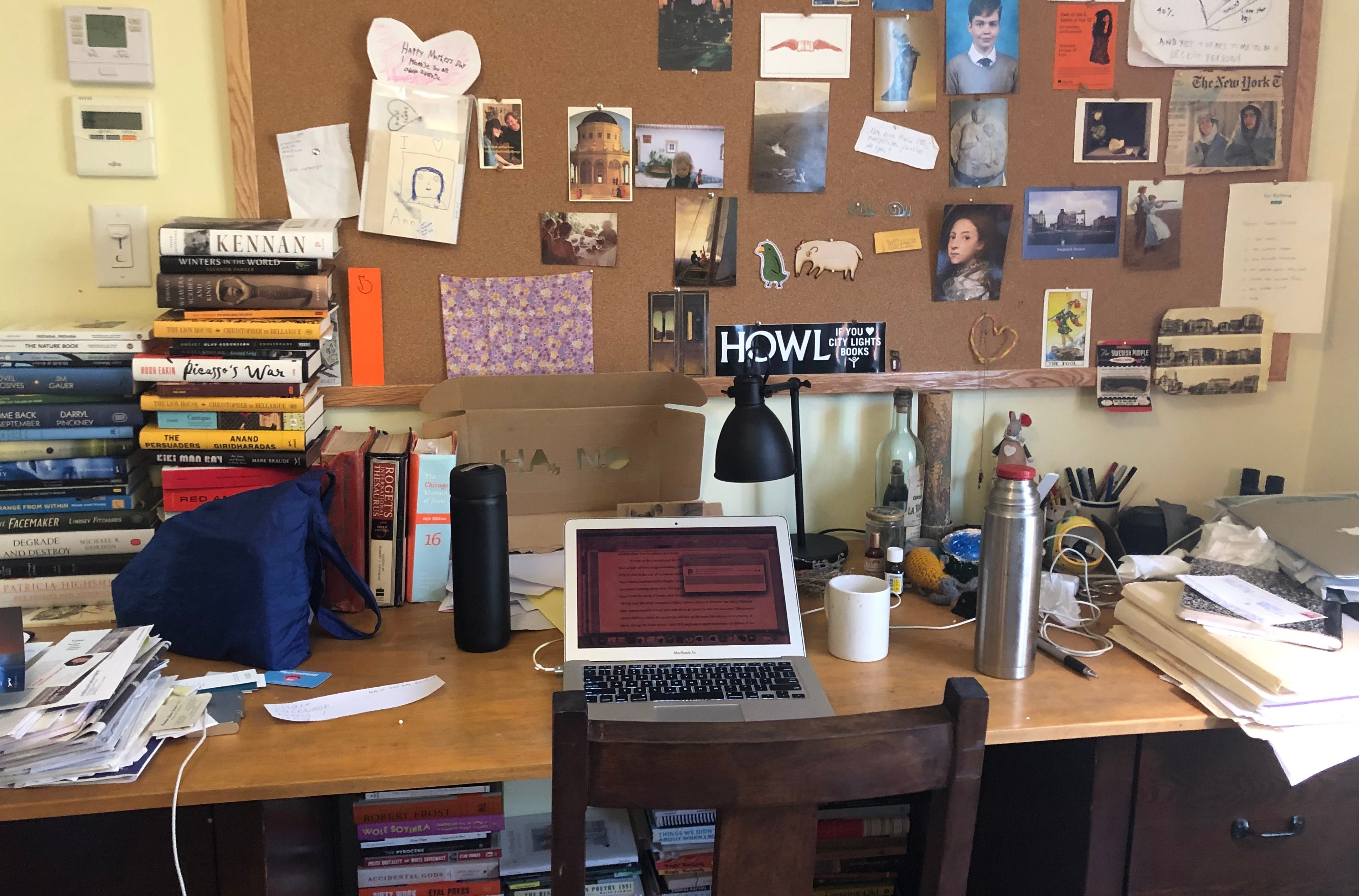The image depicts a cluttered home office or student's desk, likely in a dorm room, set against a tan-colored wall. The desk itself is a long, light brown wooden surface and features a dark brown chair. A small laptop sits in the center, flanked by a white mug and a black thermos on the left, while a silver thermos with a red lid is on the right. Behind the laptop stands a black desk lamp. To the right side of the desk, there's a noticeable accumulation of folders, papers, and several cords, as well as a cup full of pens. Further right, an empty wine bottle can be seen. On the left side of the desk are two stacks of large books. An assortment of envelopes for mail spreads across the desk area. Above the desk, a large cork board is mounted on the wall, filled with a chaotic mix of pinned photographs, postcards, newspaper clippings, bumper stickers, invitations, to-do lists, and drawings, adding to the busy and personalized atmosphere of the workspace.